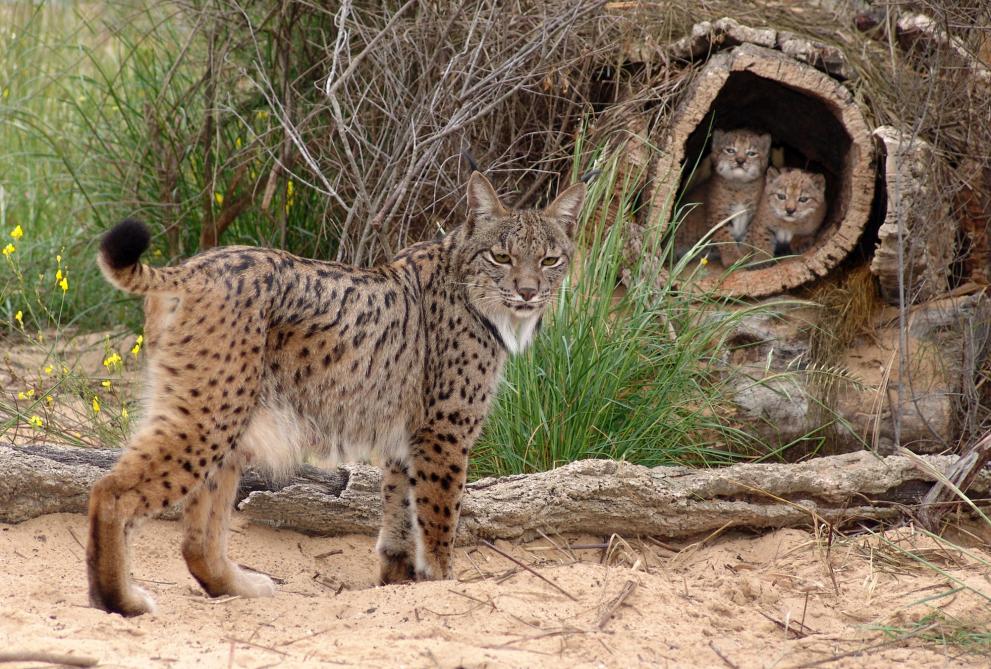In this captivating outdoor scene set in the wild, a striking bobcat with light brown fur adorned with black speckles and longer black markings around its belly stands staunchly on the sandy, beige-colored ground to the left. The bobcat's head, which looks like an enlarged domestic cat's face complete with a white "beard," is turned towards the camera, creating an engaging connection with the viewer. Its body language exudes a regal stance, showcasing its long legs and black-tipped tail.

On the right side of the image, the upper right-hand corner hosts a hollowed-out log that serves as a cozy hideaway for three adorable bobcat cubs. These tiny, brownish-furred cubs, bearing white chins and bellies, gaze curiously out from their wooden sanctuary. One cub looks down towards its guardian, while another stares directly into the camera with a somewhat smug expression.

Surrounding this family tableau, the environment is a tangle of rocks, sticks, dead leaves, and trees, interspersed with patches of wild, tall grass and overgrown weeds. A long, horizontal tree branch extends across the bottom portion of the image, accentuating the natural setting. The upper left-hand corner is a burst of greenery, completing this vivid portrait of wild beauty and familial bonds.